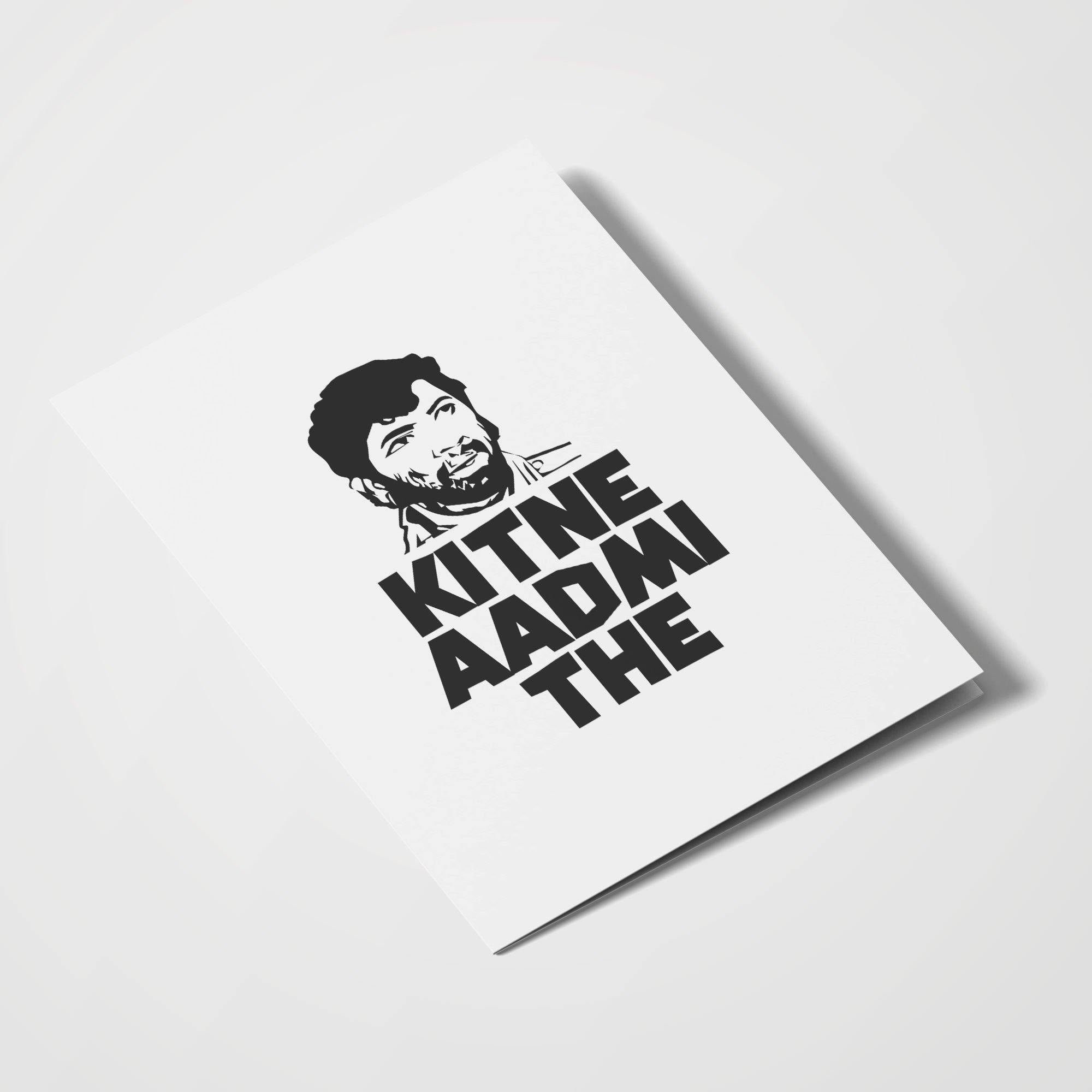This image features a small, white pamphlet set at a slight diagonal angle. The pamphlet is rectangular in shape and predominantly white. It contains black text in an unknown language that reads, "KIT-NEY AD-ME THE." Positioned above the text is a black-and-white silhouette of a man's face. The man has a beard and a scruffy appearance, and appears to be wearing a shirt, although only his head and neck are visible. The entire pamphlet is set against a clean, white background.